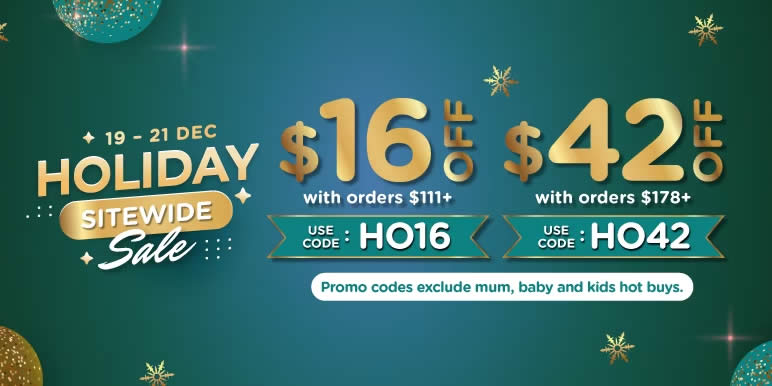**Holiday Sale Announcement**

From December 19th to the 21st, enjoy a festive site-wide sale with special discounts! The background features a charming greenish-blue hue adorned with images of ornaments and gold snowflakes, creating a winter wonderland ambiance.

**Promotions:**
- **HOLIDAY** (all-caps in gold-bordered text) is prominently displayed.
- **SALE** written in elegant cursive white text beneath.

To the right of this, centered on the flyer:
- **$16** off orders of $111 or more with code **HO16**. This text is presented within a blue banner resembling a raffle ticket.
- **$42** off orders of $178 or more with code **HO42**. This discount is highlighted in large gold text with the qualifying amount listed in white.

**Additional Information:**
- A white bubble at the bottom states: Promo codes exclude mom, baby, and kids' hot buys, written in green text.

Take advantage of these fantastic deals and make the season even brighter!